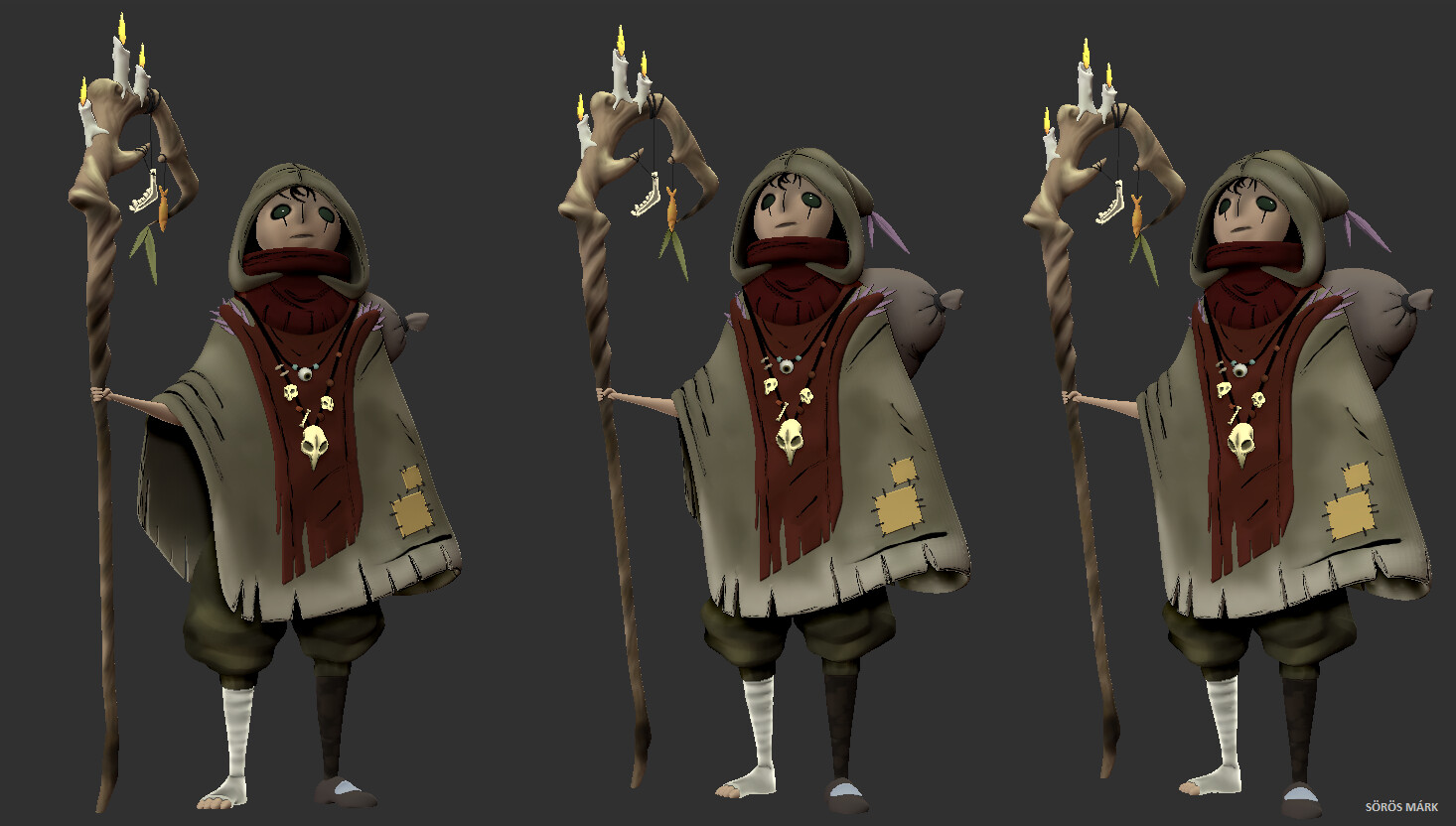The image features three nearly identical side-by-side illustrations of an animated character adorned in a long, hooded cloak that reaches just above their knees. The character, whose gender is ambiguous, holds a long staff in their right hand, topped with three burning, melting candles. Their right foot and calf are bandaged, and their left leg stands face-forward and unwrapped. They wear a large poncho accented with a red scarf, a necklace with various trinkets, and display dark eyes. The cloak has noticeable yellow patches on the lower right side as well as some skull adornments. Additionally, the character carries a knapsack attached to their back.